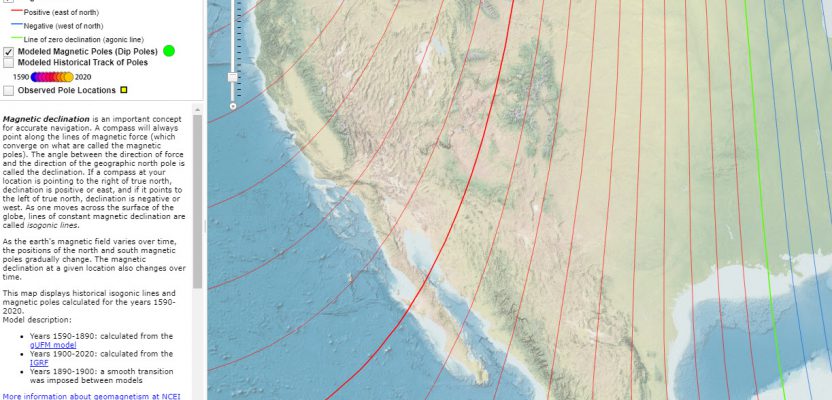This image is a detailed map focusing on part of the United States, including the West Coast by California and part of Mexico, overlaid with lines indicating magnetic movements. The lines, which are red, green, and blue, represent different aspects of the magnetic field: red for positive, blue for negative, and green for the zero line. On the left-hand side of the image, there is a sidebar providing explanations about the magnetic movements, the movement of the magnetic poles over time, and historical calculations. The key on the upper left explains that the lines depict modeled magnetic poles, model historic track poles, and observed pole locations. Below the key, there are bars showing different colors and three paragraphs discussing magnetic declination, navigation, and the Earth's magnetic field. The image is a cropped screenshot from a website, not showing the full page. At the bottom of the image, there is a blue bolded statement directing viewers to find more information about geomagnetism at the NCEI.